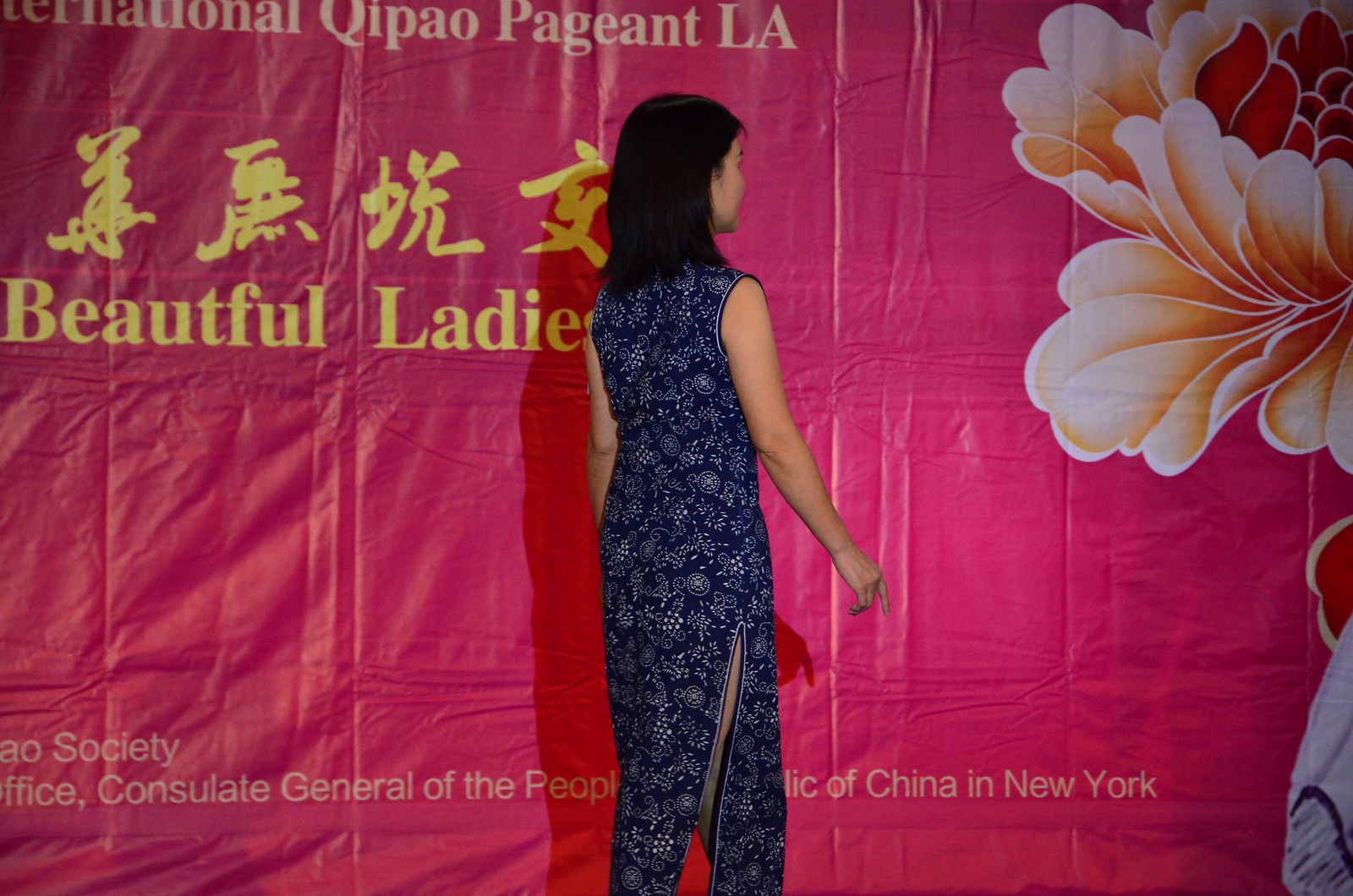The image features a young woman standing on a stage, wearing a traditional Chinese blue sleeveless qipao dress adorned with intricate beadwork, including a white floral print and an ornate pattern of swirls and circles. The dress also has a stylish split going up the side. She has shoulder-length dark black hair and is facing towards the right side of the image. The stage backdrop is pink and includes text that reads "International Qipao Pageant LA" with additional Chinese characters. There's a prominent gold text stating "Beautiful Ladies" and smaller text at the bottom indicating "Consulate General of the People's Republic of China in New York." The right side of the backdrop also features an illustrated flower.